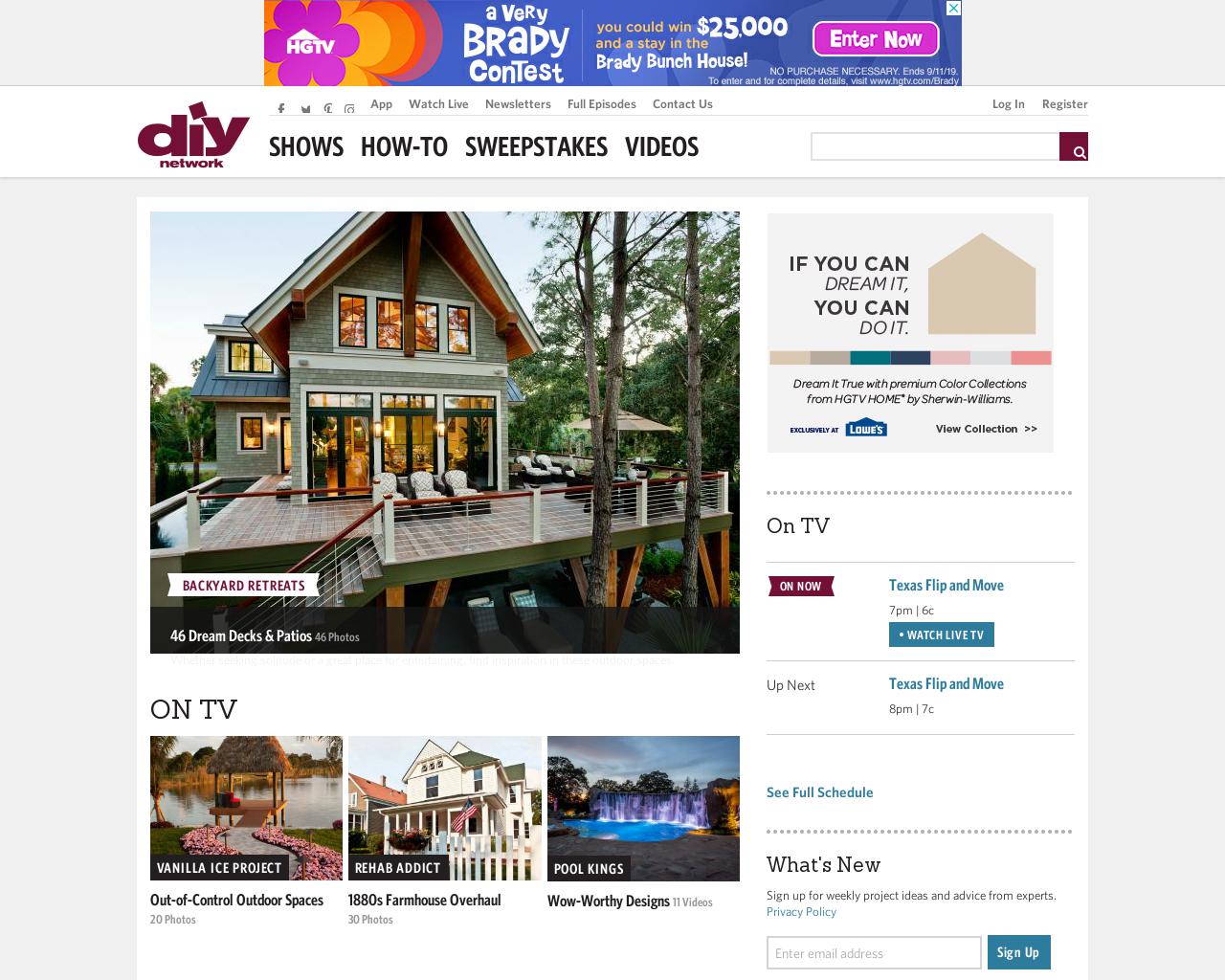This is a detailed description of a screenshot taken from the DIY Network website, illustrating the various sections and content available for viewers. 

The top banner prominently features an HGTV contest promotion with a chance to win $25,000 and stay in the iconic Brady Bunch house. This banner is flanked by social media links to Facebook, Twitter, Pinterest, and Instagram. Additionally, there are options to access features such as "Watch Live," newsletters, full episodes, contact information, and user account management (login/register).

Below the banner, the main navigation menu includes categories like "Shows," "How-To," "Sweepstakes," and "Videos." A featured image showcases a beautifully designed house titled "Backyard Retreats," accompanied by a subheading that reads "46 Dream Decks and Patios." Beside this is an advertisement for "HGTV Home by Sherwin-Williams," promoting their premium color collections.

The current and upcoming shows are listed, with "Texas Flip and Move" airing at 7 PM/6 Central, followed by another episode at 8 PM/7 Central. Thumbnails of popular shows such as "The Vanilla Ice Project" and "Out of Control Outdoor Spaces" with 20 photos each, "Rehab Addict: 1880s Farmhouse Overhaul" with 30 pictures, and "Pool Kings: Wow-Worthy Designs" with 11 videos are also displayed. An option to "See Full Schedule" is linked for more detailed programming information.

The layout encourages users to sign up for additional features and links to a privacy policy, emphasizing the website's commitment to user data protection. Overall, the website layout highlights a variety of DIY projects, TV shows, and interactive content, while also promoting contests and sponsored products.